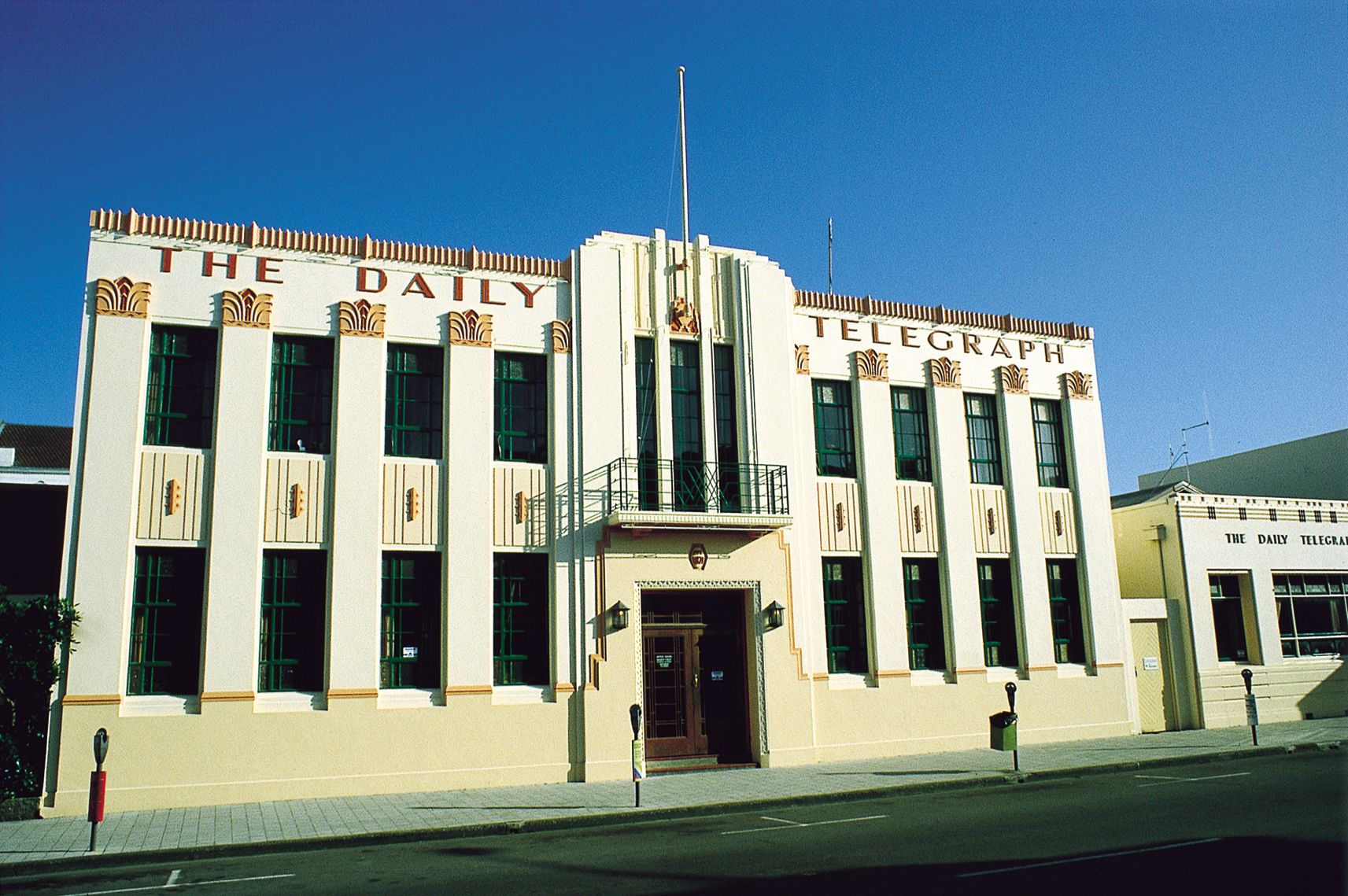The image showcases a two-story building with a prominent sign reading "The Daily Telegraph" at the top, with "The Daily" on the left, a central section that protrudes outward, and "Telegraph" on the right, all in brown, capital letters. This building is primarily tan with yellow accents and intricate yellow and red designs at the top. The facade features eight windows on each side, divided by white vertical columns, with four windows on the top and bottom floors on each side. Central to the upper floor is a small balcony with a black banister, behind which are three tall, slender windows. Below the balcony, the entrance comprises double wooden doors with glass panels, set back in a square cutout flanked by two sconce lights. The gray, stone-tiled sidewalk in front of the building features several parking meters, and the street is dark-colored with white parking lines along the curb. Adjacent to the main structure, on the right, stands a shorter, plainer building also bearing the name "The Daily Telegraph." The photo captures a clear, sunny day with a vibrant blue sky.